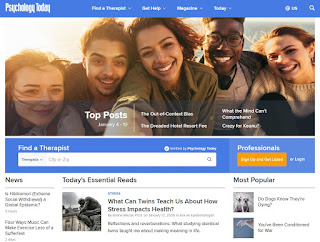Screenshot of a Psychology Today website page displayed on a computer monitor. A bright blue banner stretches horizontally across the top, featuring "Psychology Today" in bold white letters on the left, followed by menu options in white letters: "Find a Therapist," "Self-Help," "Magazine," and "Today." In the upper right-hand corner, there's an icon resembling a clock (though too small to decipher) and a white magnifying glass symbolizing search functionality.

Below the banner is a prominent site-wide image of five young adults, possibly in their late 20s to early 30s, crowded together as if taking a group selfie, all gazing directly at the camera. The left side of this image is overlaid with "Top Posts" in white text, while additional white text is present on the right side but is too small to read.

Further down is another blue banner, this time with a white search bar on the left for locating a therapist, accompanied by an orange rectangular button on the right, which is again marked with white text that's too small to read. Above the search bar, the word "Find a Therapist" is visible, and "Professionals" is seen above the orange button.

At the bottom of the page, three sections are labeled: "News" on the left, "Today's Essential Reads" in the center, and "Most Popular" on the right. The paragraphs beneath these headers contain text that is too small to discern. A legible sub-headline in the center reads: "What Can Twins Teach Us About How Stress Impacts Health?" To its left is an image of the statue, "The Thinker." Under the "Most Popular" section on the right, there is an image of two dogs and another below it depicting the ocean.